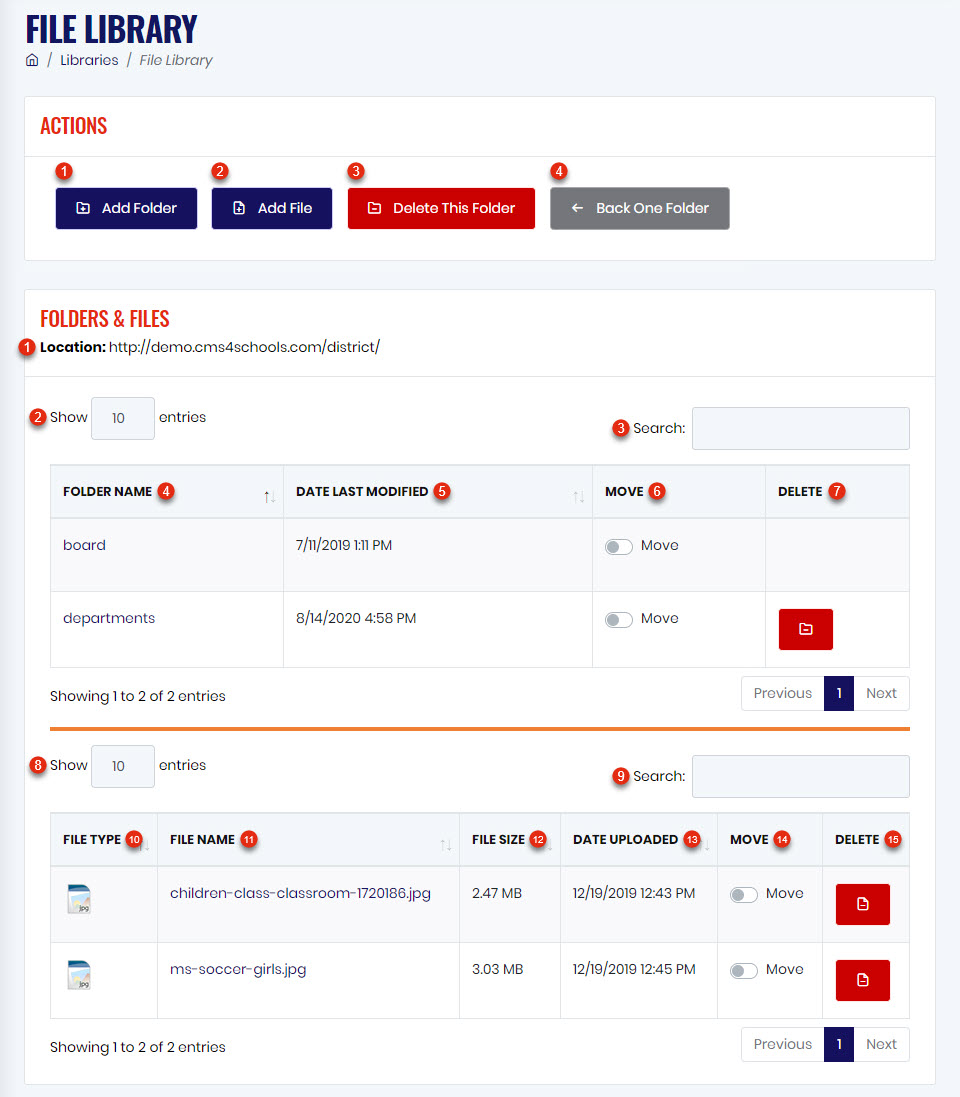The screenshot showcases the interface of a website called "File Library," presented with a blue-themed design. Multiple icons are aligned at the top, including "Home," "Library/Home," and "Library/File Library," guiding the user through different sections of the platform. Below this navigation bar, the interface is divided into several distinct sections with labeled boxes.

The first box, prominently featuring red text and labeled "Actions," comprises four buttons:
1. "Add Folder" - Buttoned in dark blue with white text.
2. "Add File" - Also in dark blue with white text.
3. "Delete This Folder" - Highlighted with a red box and white text, accompanied by a folder icon.
4. "Back One Folder" - A gray button with an embedded back arrow icon.

The second, larger box, labeled "Folders and Files" in red, further organizes the content:
1. "Location" - Contains a hyperlink, presumably directing the user to the current file directory.
2. "Show 10 entries" - Features a customizable drop-down menu displaying '10' entries.
3. "Search" - Includes a search bar for locating specific files or folders.

Following these labels, a table is structured to list the files and folders within the library:
- The header row lists: "Folder Name," "Date Last Modified," "Move," and "Delete."
- The table appears to be a four-column by three-row grid, indicating space for multiple entries.

Beneath this section, another, larger table presents additional entries. This second table is six rows by three columns, offering an expanded view of the folder and file details.

Overall, the screenshot reveals an organized, user-friendly interface designed for efficient file management within the "File Library" website.